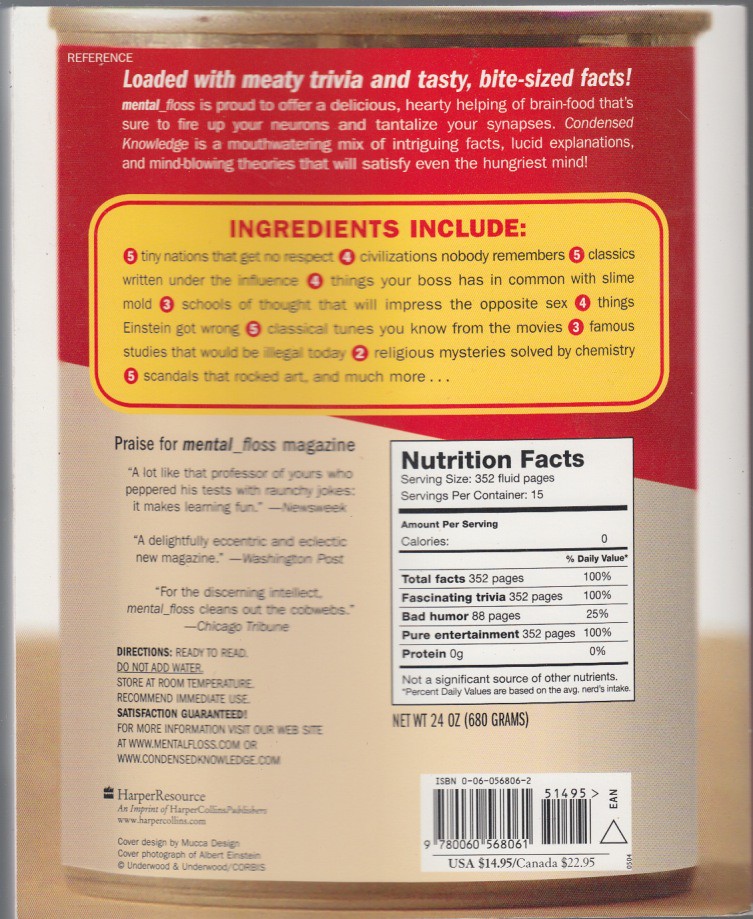This image captures the back cover of a book designed to mimic the style of a Campbell's Soup label, featuring a playful and creative layout. The cover intriguingly presents the book as a can of soup, with the title "Condensed Knowledge" and the tagline "loaded with media trivia and tasty bite-sized facts." It has a computer-generated feel, adding to its unique charm.

The description promotes the book as "a delicious, hearty helping of brain food that's sure to fire up your neurons and tantalize your synapses." It highlights the content as "a mouth-watering mix of intriguing facts, lucid explanations, and fascinating theories."

The book's "nutritional information" humorously states the volume as 352 pages of "Pure Entertainment," with 80 pages of "Bad Humor" and 0 grams of protein. The "directions" advise readers to "ready to read, do not add water," and suggest storing at room temperature with immediate use recommended. Additionally, it guarantees satisfaction.

A barcode is present, alongside the publisher's information, Harper Resource. The price is listed as $14.95 in the United States and $22.95 in Canada.